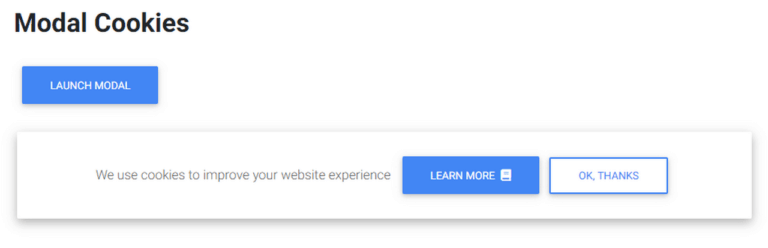The image depicts a partial screenshot of a cookie consent message commonly found on websites. At the top, there's a heading that reads, "Model Cookies," with "Model" spelled with an 'A.' Below the heading, there is a blue button labeled "Launch Model." The main body of the message states, "We use cookies to improve your website experience." Beneath this, there are two buttons: a blue button that likely says, "Learn More," and a white button with blue text that possibly reads, "Okay, Thanks." The visual design includes blue and white text, as well as blue and white borders, adding to the clarity and aesthetics of the message. Notably, there is no cursor present in the image, indicating that it is a static screenshot rather than an interactive element.